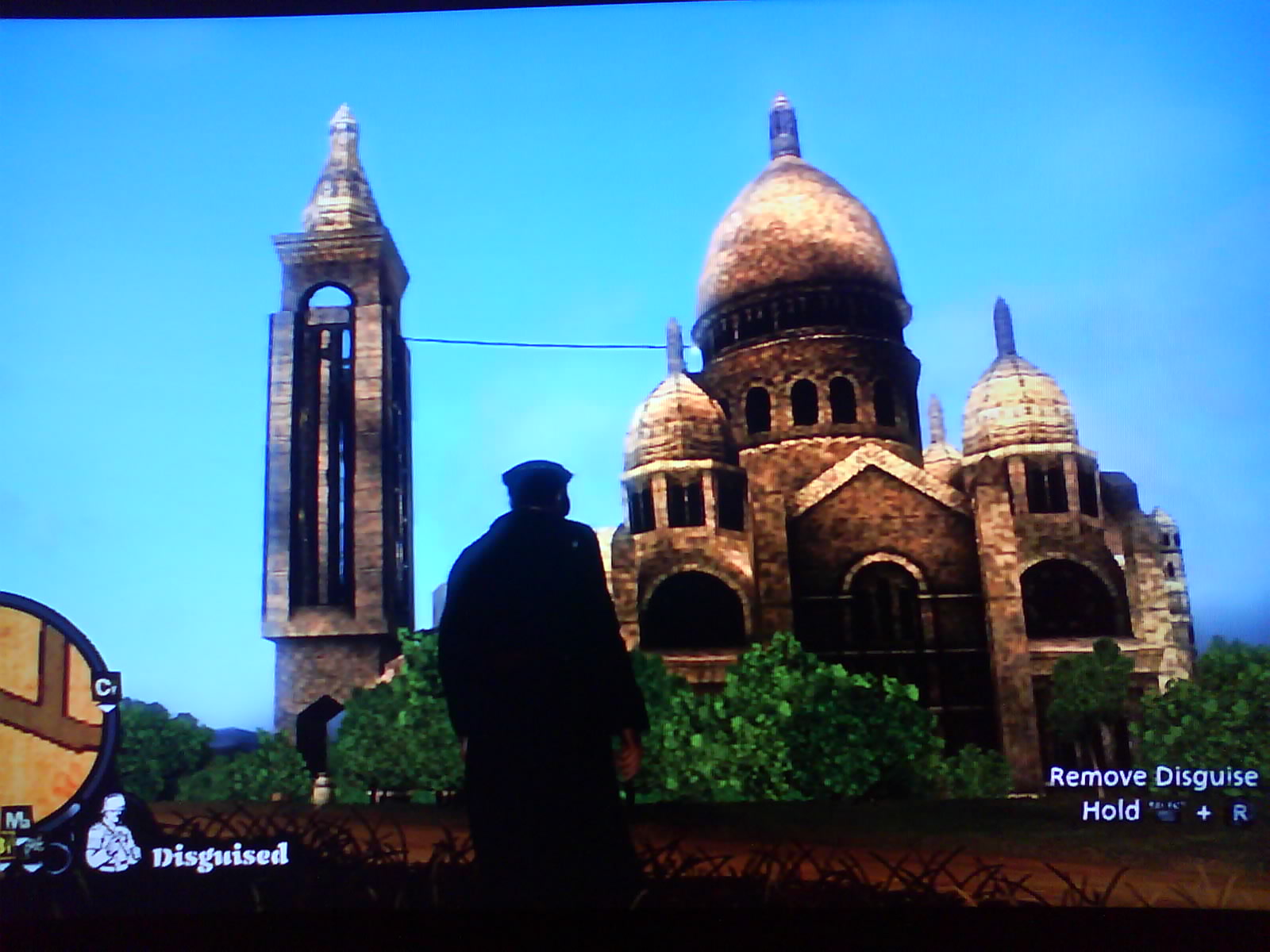In the image, we see a vivid screenshot from a video game that features an intricately detailed mosque-like structure prominently in the center. The mosque, showcasing a blend of gold and deep brown hues, boasts several dome-shaped roofs with ornate pointy pillars on top. It is surrounded by green plants at its base and connected by a cable to a rectangular brown building on the left. The sky in the background is a brilliant blue with a hint of clouds. 

A man dressed in a long black coat and cap, facing away from the viewer and towards the temple, stands in the center of the frame, casting a silhouette in the shadows. On the bottom left corner of the screen, there is a circular map with a schematic, white drawing of a soldier's head and the word "disguised" written in white. On the bottom right corner, white text reads "remove disguise" with "hold" partially visible below it. Black plants can be seen at the bottom of the image, adding to the overall depth and detail of the scene.